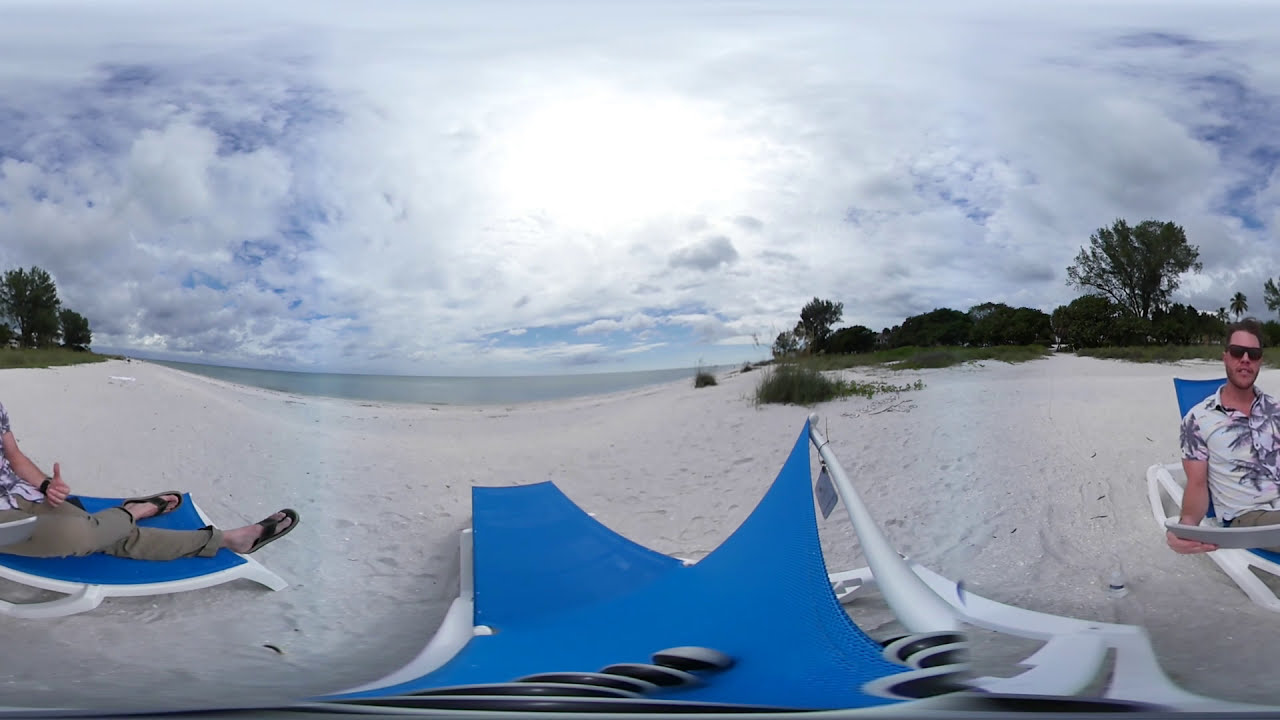The image depicts a man sitting near the shoreline on a large, relatively empty beach. He is seated on a blue lawn chair with a white frame, wearing a white aloha shirt adorned with a tropical palm tree pattern, sunglasses, khaki pants, and flip-flops. The image seems to be a panoramic or 360-degree view, given the distorted and repeating elements. The man's upper body and newspaper appear on the right, while his legs reappear on the left. The beach sand is flat and white, and the background features calm, dark grayish-blue ocean waters, surrounded by low grasses, trees, and shrubs. The sky is overcast but allows some sunlight to filter through the clouds, adding to the serene daytime atmosphere.